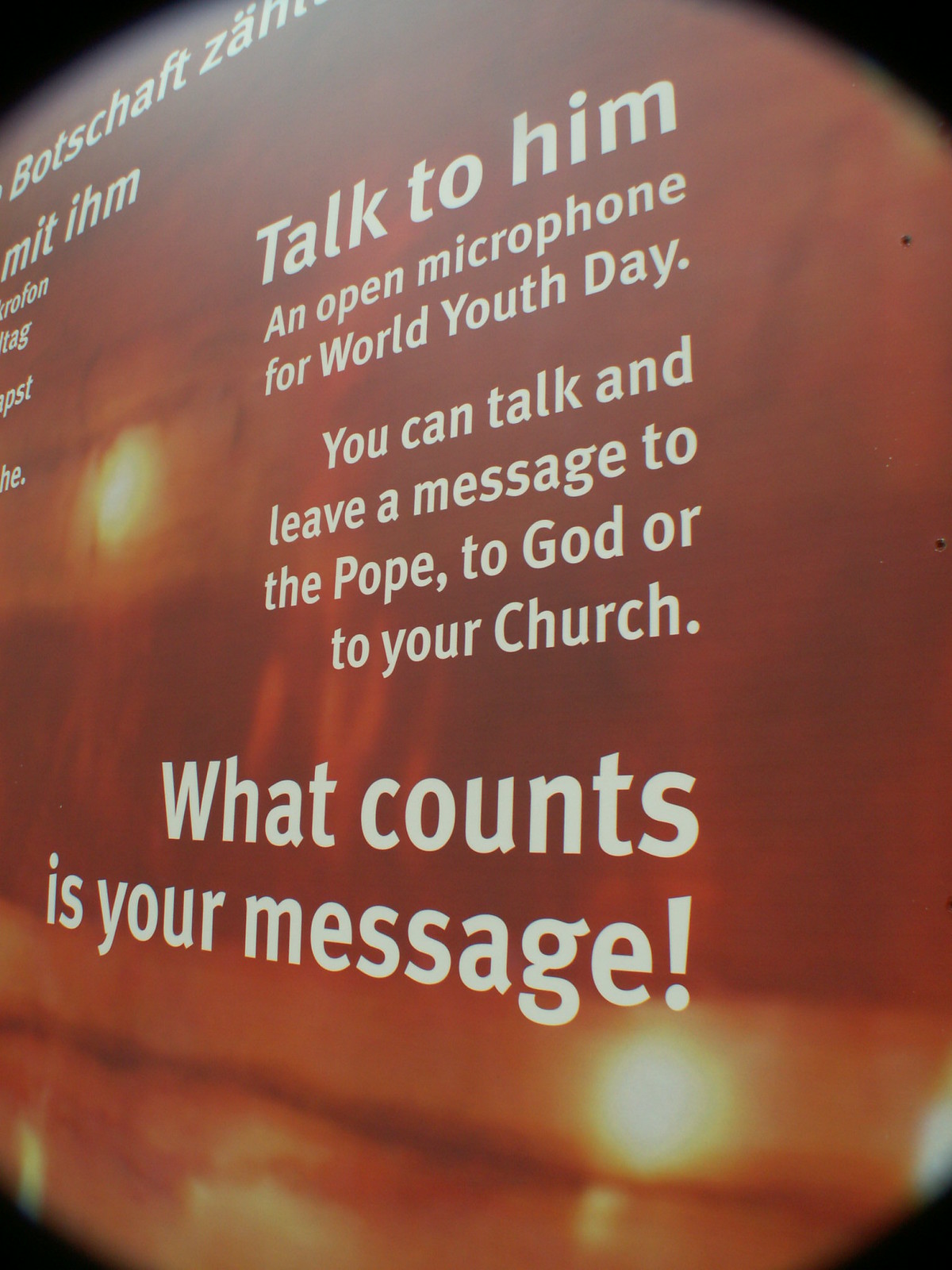The image captures a vivid, reflective surface displaying a prominent religious message, possibly formatted as a poster or PowerPoint presentation. The background showcases a dramatic reddish-orange sunset over water, creating an eye-catching vignette effect with black corners. Central to the composition is a column of easily readable white text, which reads: "Talk to Him, an open microphone for World Youth Day. You can talk and leave a message to the Pope, to God, or to your church. What counts is your message." The textual content is mirrored both in English on the right and a partially visible German version on the left. This picture is likely intended for a multilingual religious event, suggested by the dual-language presentation.